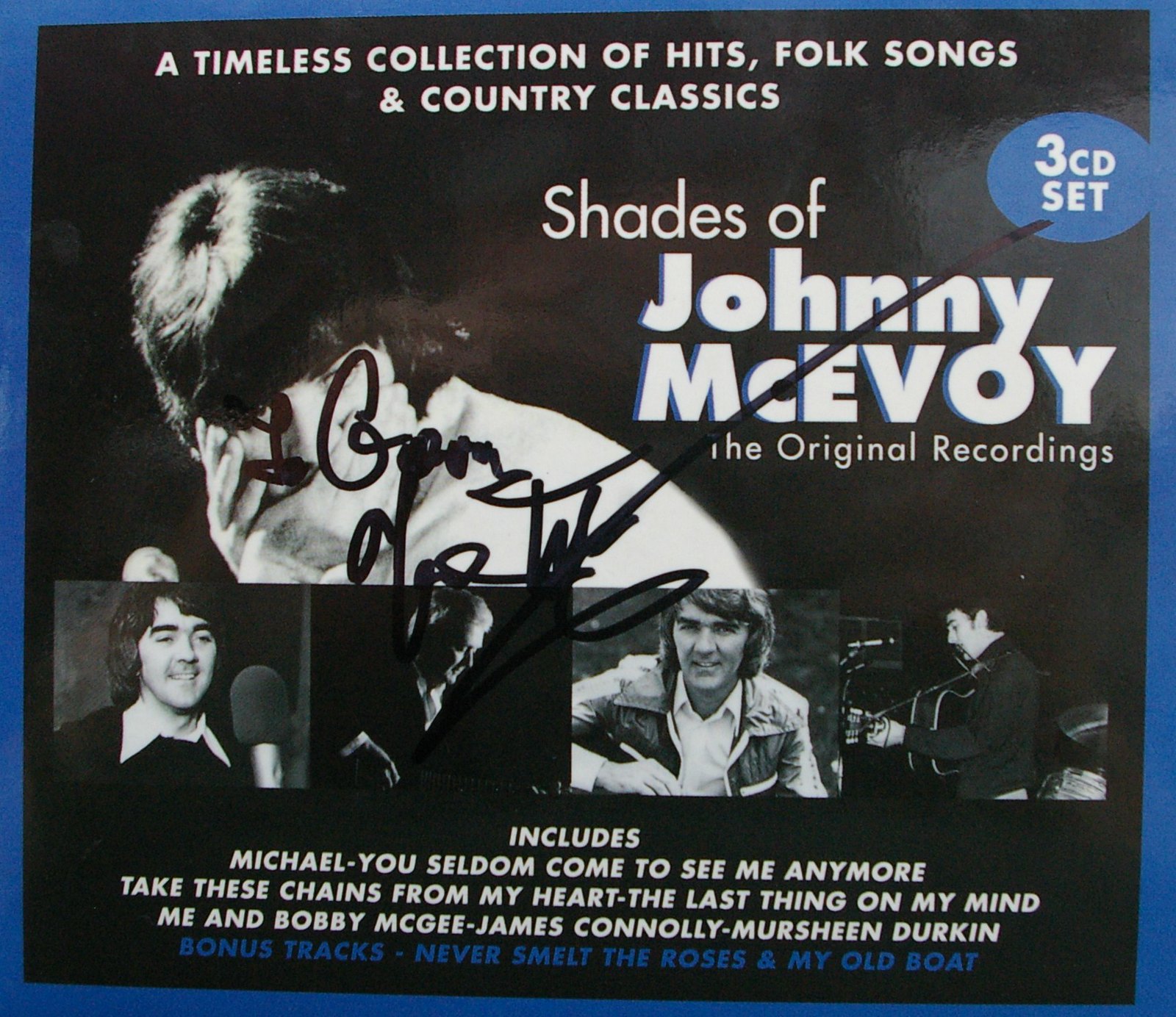The image is the front cover of a three-CD album titled "Shades of Johnny McElvoy," featuring a timeless collection of hits, folk songs, and country classics. The background is dark, with the top adorned in bold white letters proclaiming the collection's genre. Below it, in large letters on the right, it states "Shades of Johnny McElvoy," with "The Original Recordings" beneath in smaller font. The album cover includes a signature that runs across McElvoy's name, likely written with a black sharpie. A thin blue border frames the album, complemented by a blue oval in the top right corner indicating "Three CD Set."

The lower portion of the cover displays a series of black-and-white images of Johnny McElvoy playing the guitar in various outfits and settings, suggesting different times in his career. Below these images, a list of song titles is written in white, including tracks like "Michael," "You Seldom Come to See Me Anymore," "Take These Chains from My Heart," "The Last Thing on My Mind," "Me and Bobby McGee," and "James Connolly." Additionally, bonus tracks "Never Smelt the Roses" and "My Old Boat" are highlighted in blue. The overall design exudes a classic, nostalgic feel, spotlighting Johnny McElvoy's musical legacy.